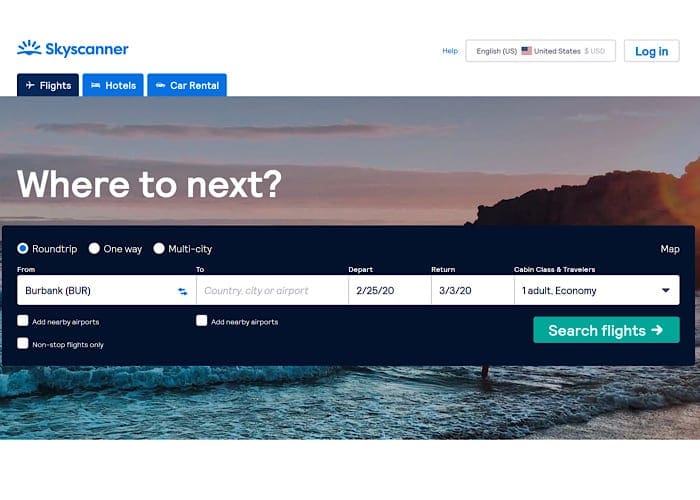This image appears to be a screenshot from a computer screen displaying the Sky Scanner website interface. At the very top, there is a prominent white border. On the upper left corner, there is a blue text that reads "Sky Scanner," accompanied by a logo depicting a blue sun with an underline. Towards the right, you see the word "Help" in blue, followed by a dropdown bar indicating "English (United States)," and a "Log in" button.

The central part of the screen is dominated by a scenic photograph. The upper segment of the picture shows a partially blue sky with scattered clouds. Below that, a thick band of clouds stretches across the image. The bottom half reveals an ocean scene with a strip of brown land jutting from the right side into the water.

In the upper left corner of the page, there are three navigation tabs labeled "Flights," "Hotels," and "Car Rental." Directly under these tabs, a header asks, "Where to next?" Below this, a large blue rectangle spans the width of the screen, indicating the user is viewing flight options. The "Round Trip" option is highlighted. Within the search fields, "Burbank" has been entered as the departure location, but no destination has been specified. The departure date is set for February 25, 2020, and the return date is March 3, 2020. The traveler is noted as one adult traveling in economy class. Beneath these details is a prominent teal button labeled "Search Flights."